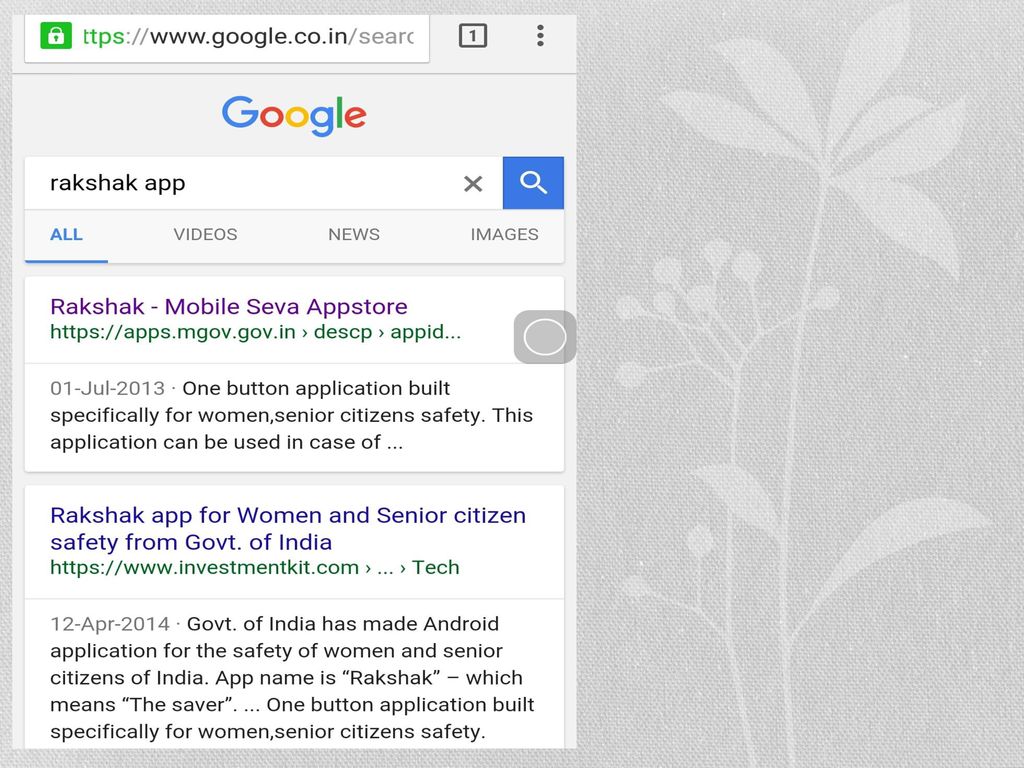The image depicts a computer screen displaying a Google search result for "Rack Shack App" (spelled R-A-K-S-H-A-K-A-P-P). The screen, which resembles a phone display, features a distinctive pattern of floral designs. On the left side, there is an overlay of the search results. The Google search interface offers options to view all results, videos, news, or images.

Two specific search results are highlighted:
1. The first result is titled "Rack Shack Mobile SEBA App Store" and links to apps.mgov.gov.in.
2. The second result is titled "Rack Shack App for Women and Senior Citizens Safety from Government of India." 

The first link directs to an app store page, describing the app as a "one-button application built specifically for William's Senior Citizen Safety." This app appears to be useful in emergency situations for women and senior citizens.